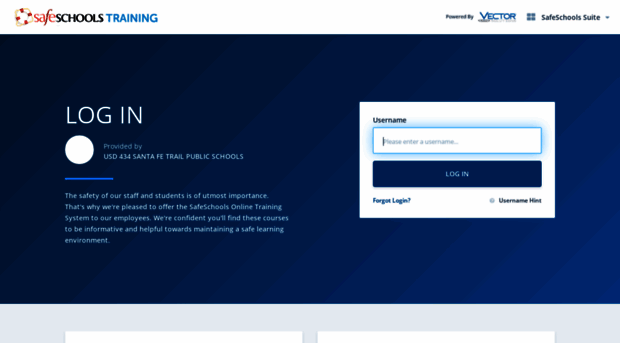This image is a screenshot of a web page that appears to be related to school or education. The top of the page features a clean white header. On the left side of the header, there is a stylized logo with the text "Safe Schools Training." The word "Safe" is written in pink lowercase letters, "Schools" in black capital letters, and "Training" in light blue capital letters. Adjacent to the logo is an icon that resembles a circle within a square, colored in shades of pink and light red similar to the word "Safe."

On the right side of the header, the text "Powered by Vector" is displayed in uppercase blue letters, with smaller, unreadable text beneath it. Further to the right, the header displays "Safe Schools Suite" in gray font, accompanied by an inverted gray triangle indicating a drop-down menu.

The background color of the remainder of the page is a gradient of blue—darker on the left and lighter towards the lower right corner. In the center, large white capital letters spell out "LOGIN." Below this is a white circle containing the text "Provided by USD 434 Santa Fe Trail Public Schools" in white font.

A brief and partially legible description beneath states, "The safety of our staff and students is of utmost importance." On the right side of the page, there is a white rectangle serving as a login area. At the top, it prompts for "Username" with a space to enter this information. Directly below, a blue rectangle with white capital lettering states "LOGIN."